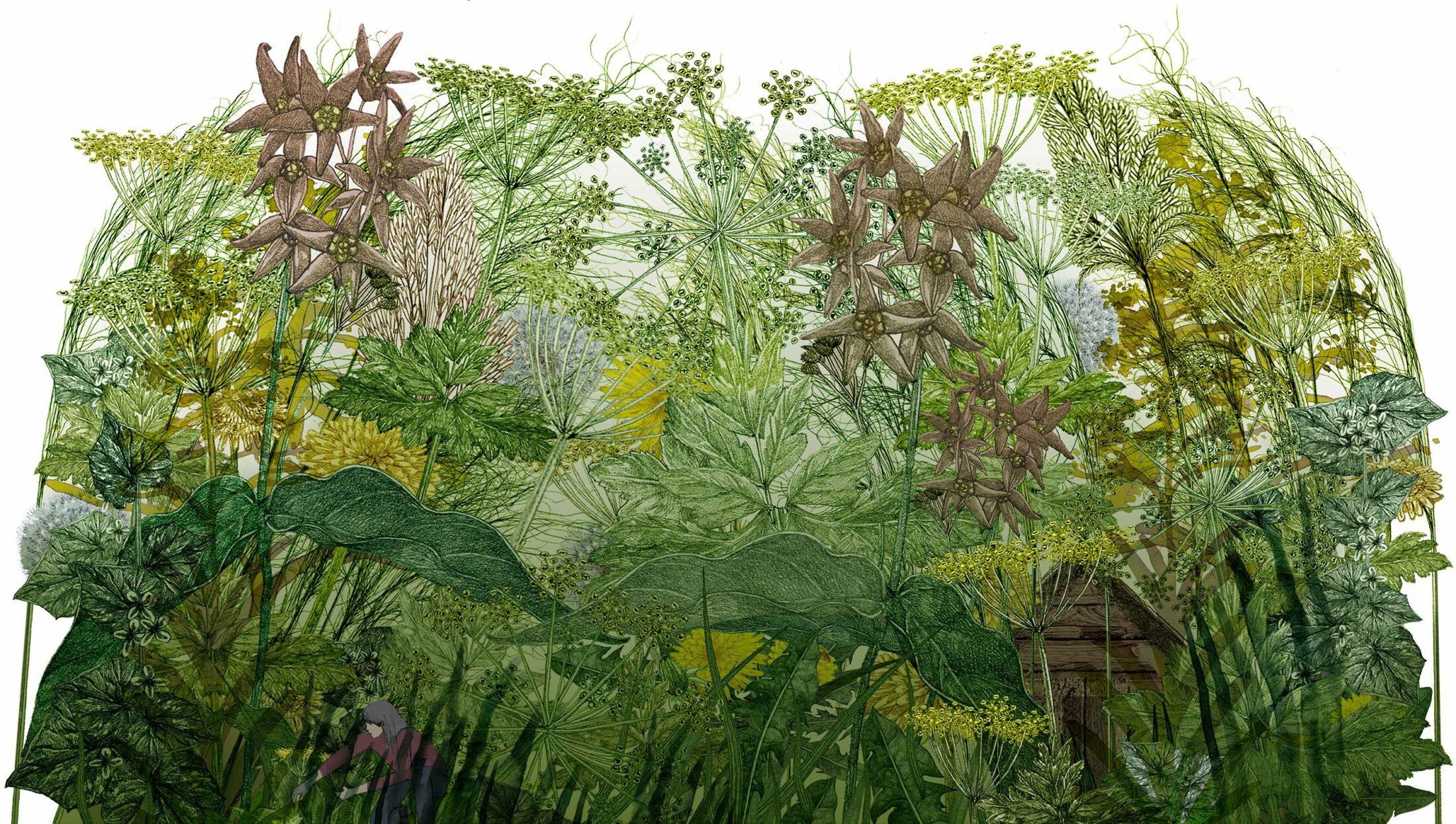This illustration depicts an outdoor scene dominated by a lush array of plants, with a lot of green hues ranging from light yellow-green to dark almost black-green, indicating a dense, vibrant greenery. From a low angle, the viewer is drawn into the verdant environment, which features an assortment of leafy plants, ferns, and scattered flowers. 

In the bottom left corner of the image, almost hidden among the foliage, a tiny, cartoon-like woman is seen in a purple shirt, bending down as if she is weeding or picking a plant. Her small stature compared to the enormous plants around her gives a whimsical feel to the image.

Amid the greenery, there are stems with golden, fluffy tops interspersed with the green foliage, as well as lighter patches of plants and air spaces as the scene ascends, giving a sense of depth. Towards the top of the image, light magenta-red blossoms add a splash of color, contrasting with the predominantly green landscape.

On the right side of the scene, partially obscured by the dense plant life, stands a brown log cabin with a triangular roof, blending naturally into the intertwined garden that surrounds it. The plants curve inward from both sides towards the center, creating a flowing composition that guides the viewer's eye through the lovely, immersive garden scene.